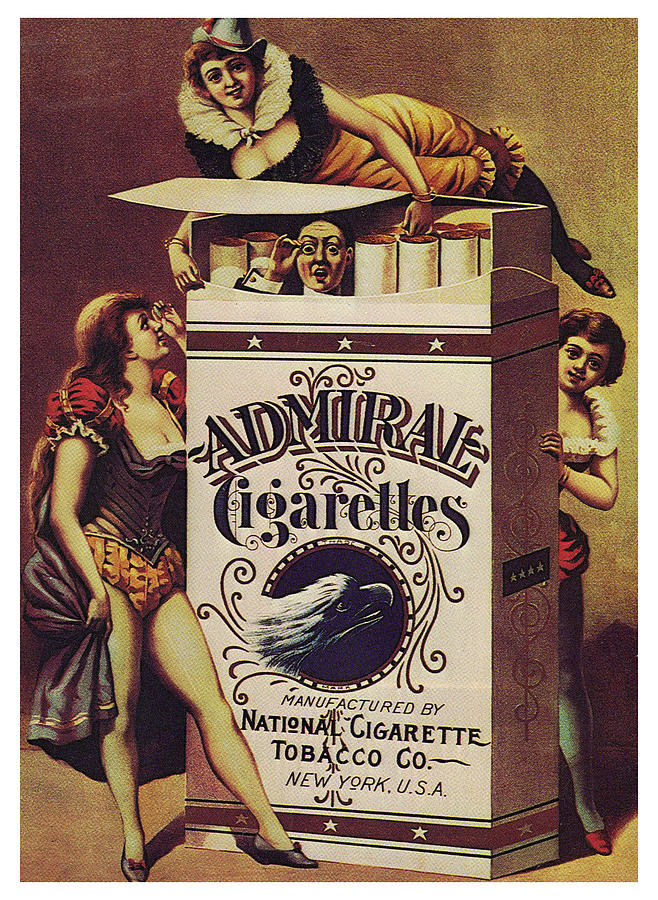This illustration is a vintage-style cigarette advertisement titled "Admiral Cigarettes," likely created by the National Cigarette Tobacco Company, New York, USA. The advertisement is a detailed color drawing, rectangular in shape and portrait in orientation, measuring approximately five inches high and three to four inches wide. 

Dominating the center is a towering white pack of Admiral Cigarettes, angled slightly with its front fully visible. Red banners adorned with white stars top and bottom the pack, while a central black circle features an eagle's head. Below the eagle, the text reads, "Manufactured by National Cigarette Tobacco Company, New York, USA." The top of the pack is open, revealing filterless cigarettes, with a man's head humorously popping out from inside. He has a surprised expression and is lifting a monocle to his eye, dressed formally with a visible cuff link.

Three scantily clad women in elaborate vintage costumes surround the cigarette pack. The woman on top reclines with a playful smile, wearing a blue top hat, ruffled pantaloons, and a white stand-up ruffled collar. To the left, another woman, dressed in short pantaloons and a blue cape, stands beside the pack looking up at the woman on top. The third woman peeks around from the right side, also in period-appropriate Gibson girl attire. The illustration's background is colored in shades of brown and gold, enhancing its nostalgic charm.